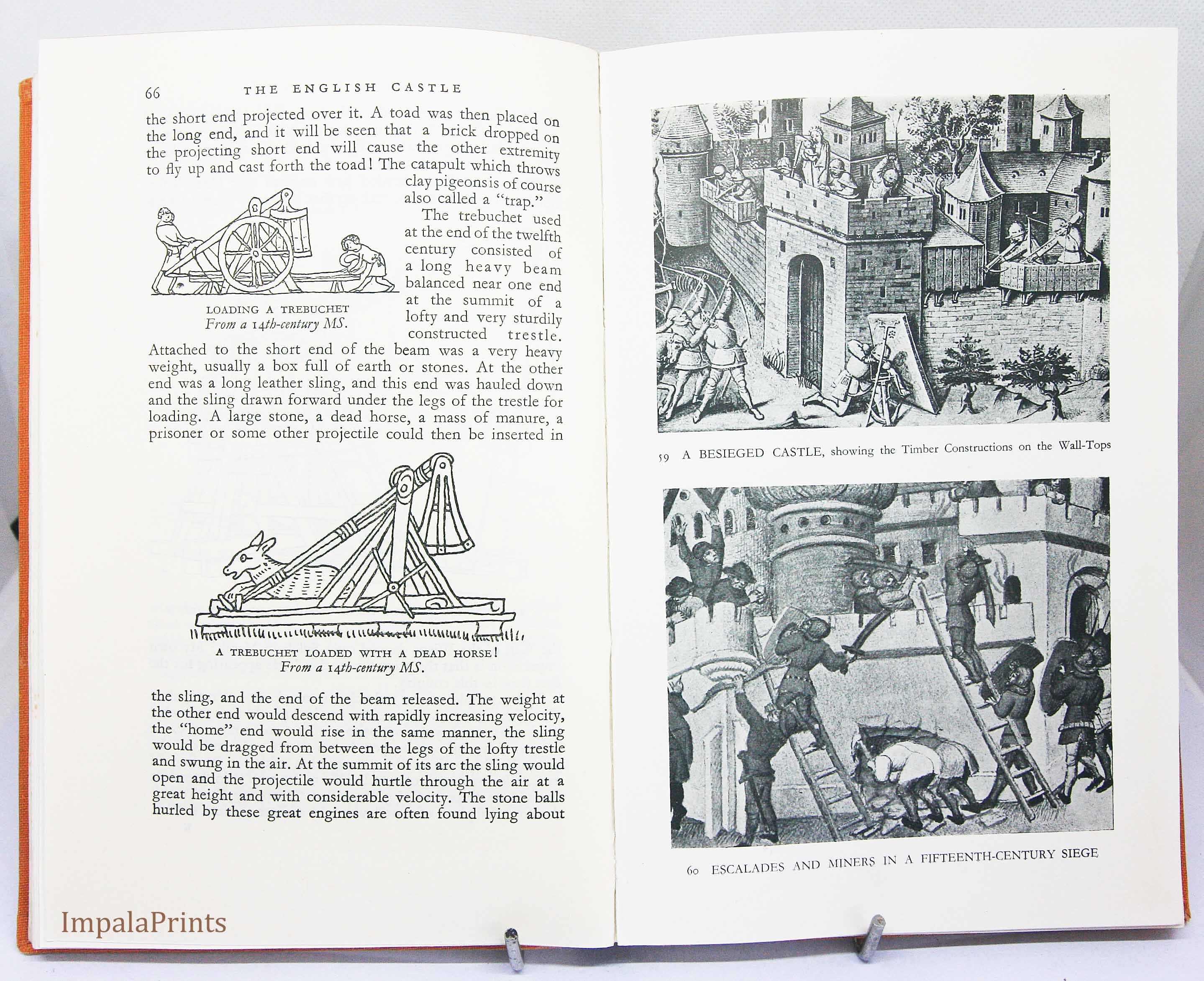This photograph captures an open book, propped up on a metal stand, showing pages 66 and 67 of a detailed text about medieval warfare, specifically focusing on sieges. The book appears to have an orange hardback cover. The left page, titled "The English Castle," has several paragraphs of text and includes two black-and-white illustrations. At the bottom left, there's a note that reads "Impala Prince."

The first illustration titled "Loading a Trebuchet," shows two figures operating a trebuchet, and the second depicts a trebuchet loaded with a dead horse. The left page provides a detailed description of how trebuchets were loaded and used during the late 12th century, emphasizing the mechanism involving a heavy beam, a counterweight, and a sling to launch various projectiles, including large stones and even dead animals.

The right page contains two large black-and-white hand-drawn illustrations that dominate the page, each with descriptive captions below. The upper illustration, labeled "A Besieged Castle," vividly portrays a chaotic scene of archers atop a castle wall shooting down at attackers, with some defenders hiding behind shields and others actively returning fire. The lower illustration, titled "Escalades and Miners in a 15th Century Siege," shows soldiers using ladders to scale the castle walls, engaged in fierce combat with defenders wielding swords and bows. Some attackers attempt to infiltrate through a breached section of the wall. The scene captures the intensity and complexity of medieval siege warfare.